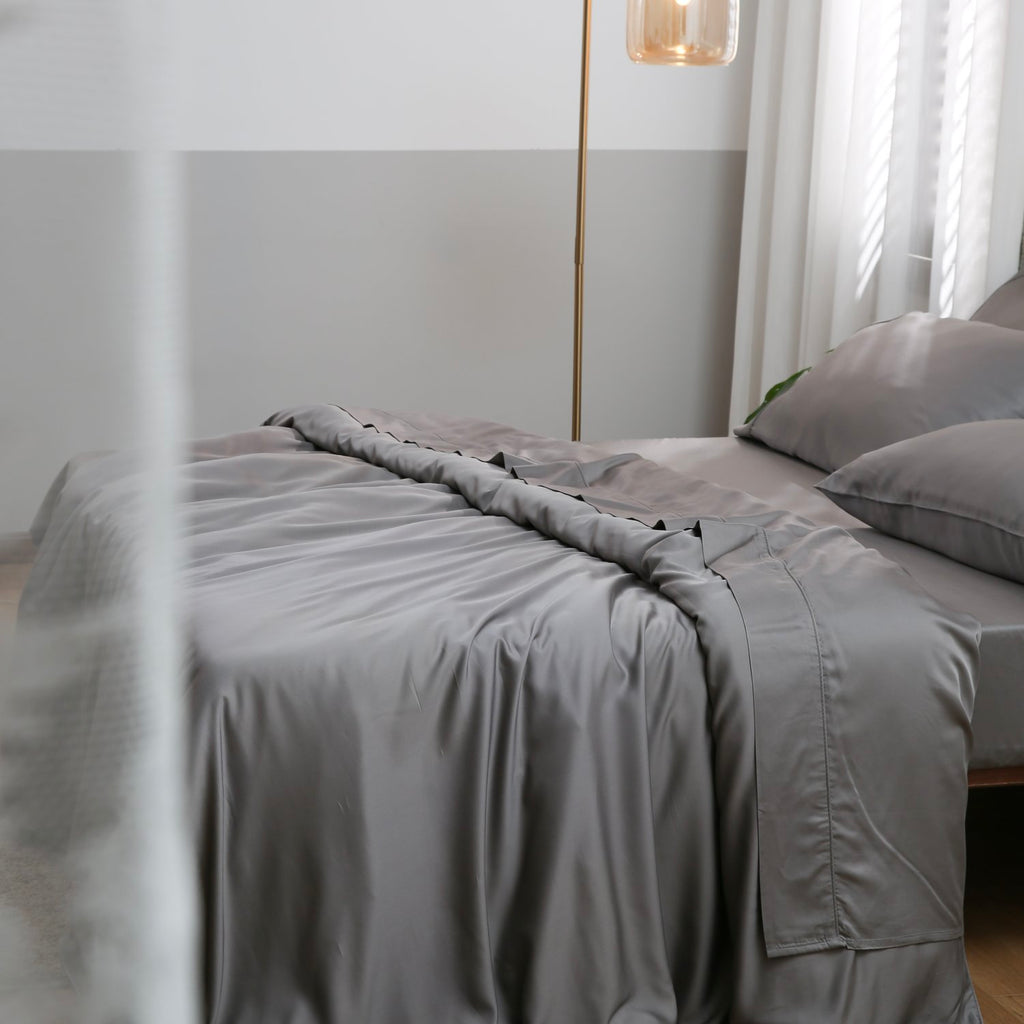The image depicts a cozy bedroom featuring a queen-size bed prominently positioned against the two-toned gray wall, which transitions from a darker shade at the bottom to a lighter hue at the top. The bed is adorned with gray, silky-looking covers, including a comforter that is pulled slightly down, with its edges touching the hardwood floor below, revealing a shiny gray sheet underneath. Puffy gray pillows rest at the head of the bed. To the far side of the bed hangs a long-necked, gold-colored lantern with a visible bulb hovering just above the bed. Adjacent to the lantern is a window adorned with sheer, white curtains, allowing light to filter through. The overall setting of the image evokes a sense of calm and subtle elegance, with the details hinting at a personal, home environment.